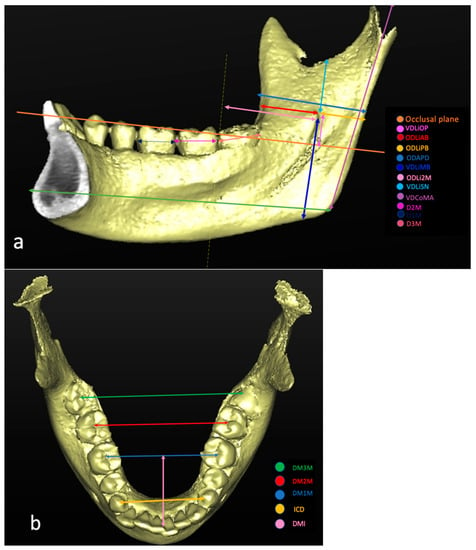The image showcases a 3D-like imaging technique or x-ray/MRI of a human jawbone, displayed from two different perspectives on a black background. The upper section, image A, presents a horizontally rectangular cross-section of the lower jaw, highlighting three molars and two canine teeth. It features multicolored dots and lines with corresponding color-coded keys on the right side, labeling parts such as the "occlusal plane". The image also has a cut section with numerous colors including orange, pink, red, tan, turquoise, dark blue, light pink, a darker red, navy, and salmon, denoting various anatomical parts or measurement points. The lower section, image B, is more square-shaped and shows a top-down view of the bottom jaw. This section includes fewer color-coded dots and lines, specifically green, red, blue, yellow, and light pink, running horizontally across the jaw, connecting and possibly identifying specific teeth or positions from left to right. A vertical light pink line divides this image down the center. Both images are detailed, with the jawbone depicted in a gold hue, and detailed annotations aiding in anatomical study.